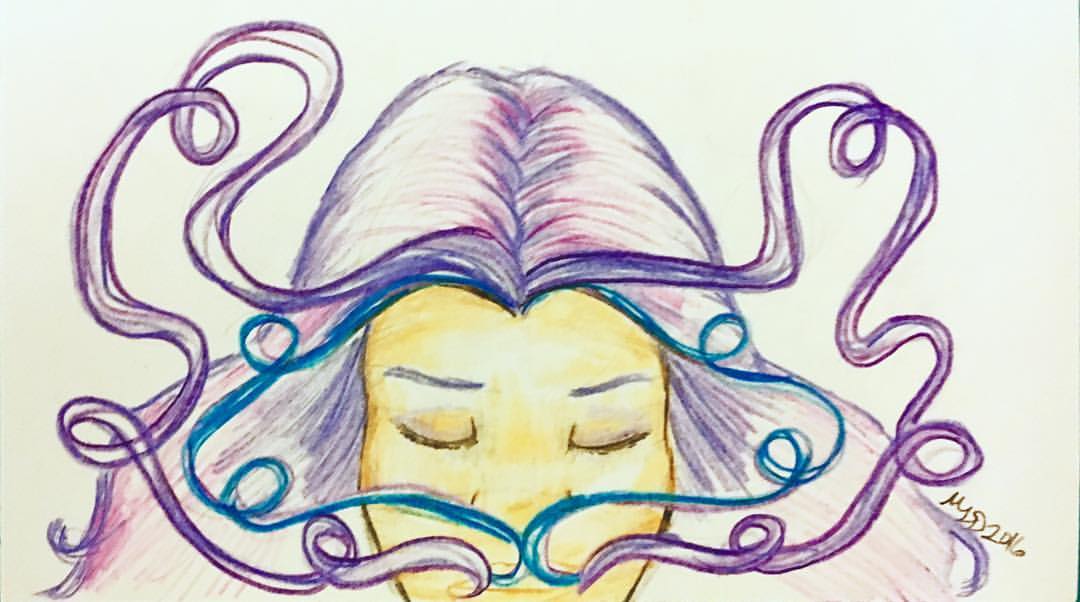This illustration, likely rendered in colored pencils or charcoals on white paper, depicts a female figure viewed from the bottom lip upward. Her head is tilted slightly downward, and her eyes are closed, giving the impression of a serene or restful state. Her skin showcases a blend of peach, orange, and yellow hues, outlined with darker shades for definition. She has thin, dark purple eyebrows, with black eyelashes highlighting her closed eyes.

Her hair is a striking feature, predominantly purple with accents of violet and hot pink near the crown, where it is parted in the middle and cascades out of view on both sides. Curly wisps of hair extend from the top and sides of her head. These tendrils are a mix of purple and white, with darker purple borders, and gracefully curl towards her nose. Additionally, thinner blue curls emerge beneath the purple strands, looping around and also converging near her nose. This intricate detail in her hair creates a dynamic and flowing appearance. The drawing is signed in brown writing at the lower right corner, adding a personal touch from the artist.